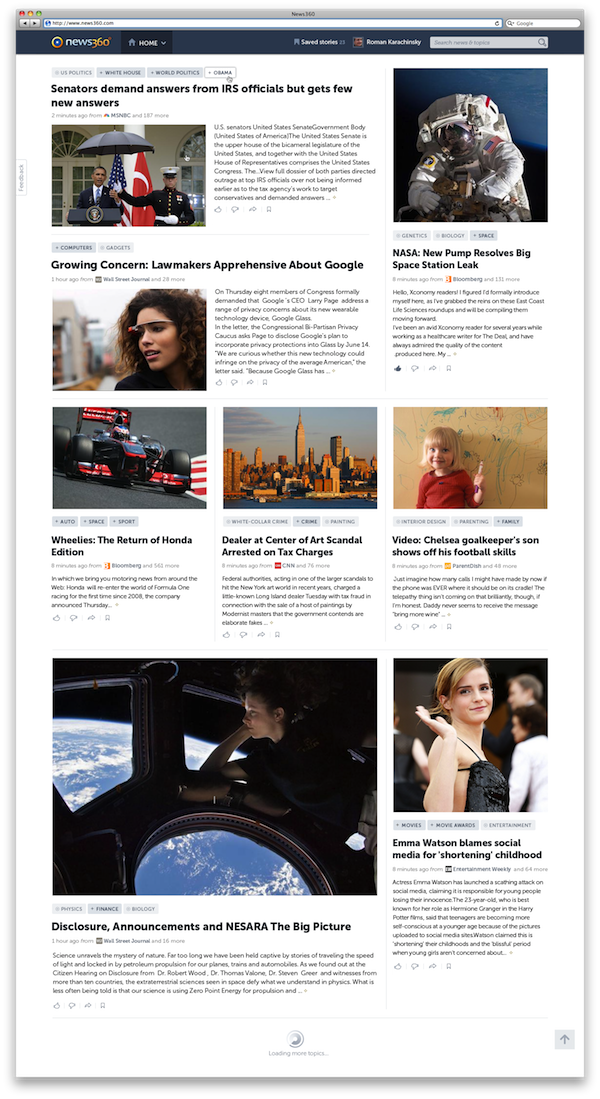The image is a screenshot displaying multiple article headlines arranged in a grid format. 

At the top, the first article reads: "Senators Demand Answers from IRS Officials But Get Few New Answers." Below this headline, another article titled "Growing Concern: Lawmakers Apprehensive about Google" is seen.

To the right, there's a headline stating: "NASA: New Pump Resolves Big Space Station Leak."

Lower in the image, three articles are lined horizontally:

1. "Wheelies: The Return of Honda Edition"
2. "Dealer at Center of Art Scandal Arrested on Tax Charges"
3. "In Video: Chelsea Goalkeeper's Son Shows Off His Football Skills"

At the bottom left of the image, an article is titled: "Disclosure Announcements: In This Era, The Big Picture." To the right, another headline reads: "Emma Watson Blazes Social Media for 'Shorting' Childhood."

The layout suggests a diverse range of topics from politics and technology to sports and entertainment.